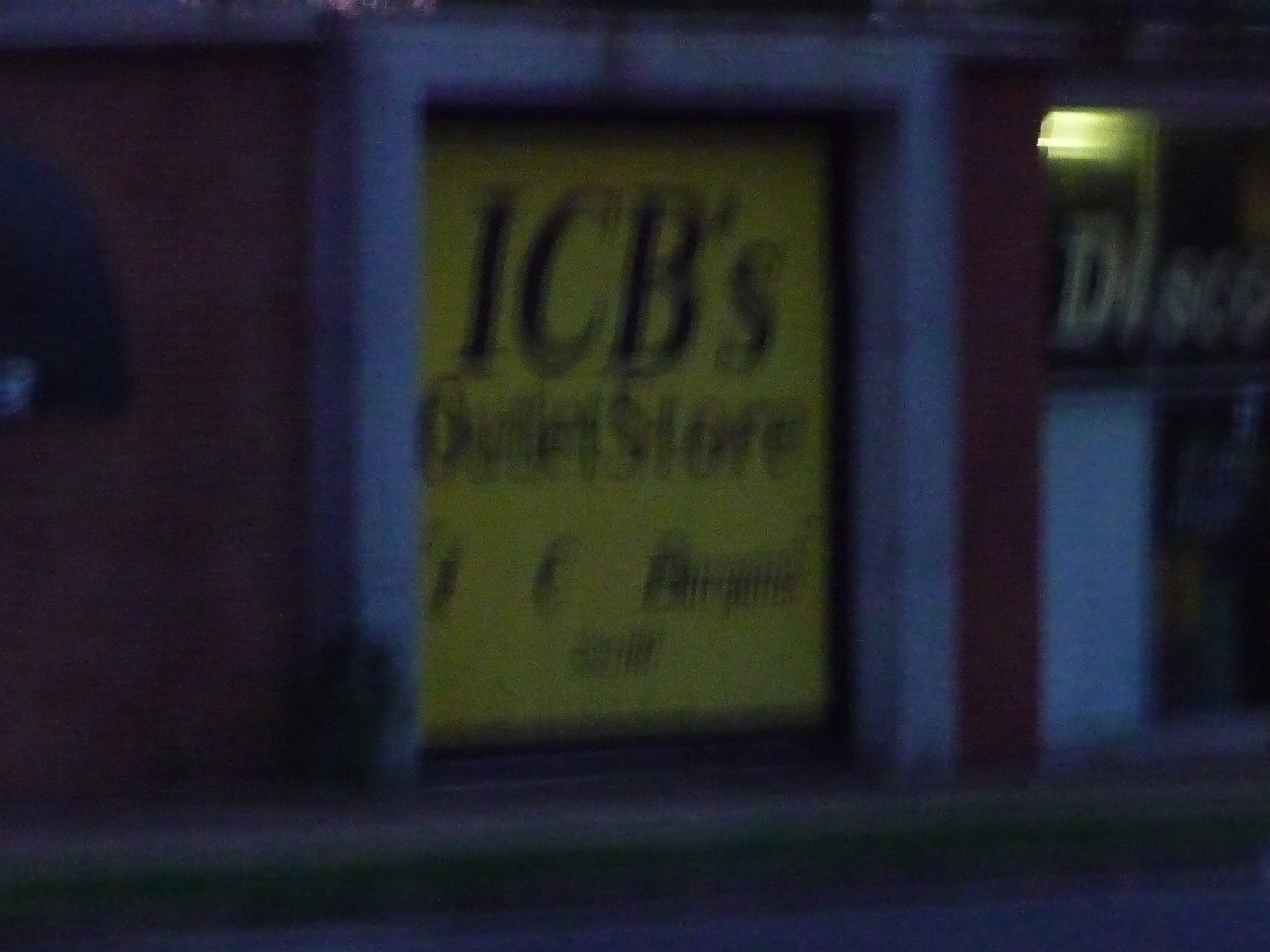This horizontally aligned photograph captures the exterior of an outlet store under poor lighting conditions, likely taken at night or during the evening. The image is noticeably out of focus and blurry. At the center, there are double doors painted yellow, prominently displaying "ICB's" in large letters above them. Below this, the words "outlet store" are written in smaller letters. A soft light emanates from the inside of the store, subtly illuminating the immediate area around the entrance.